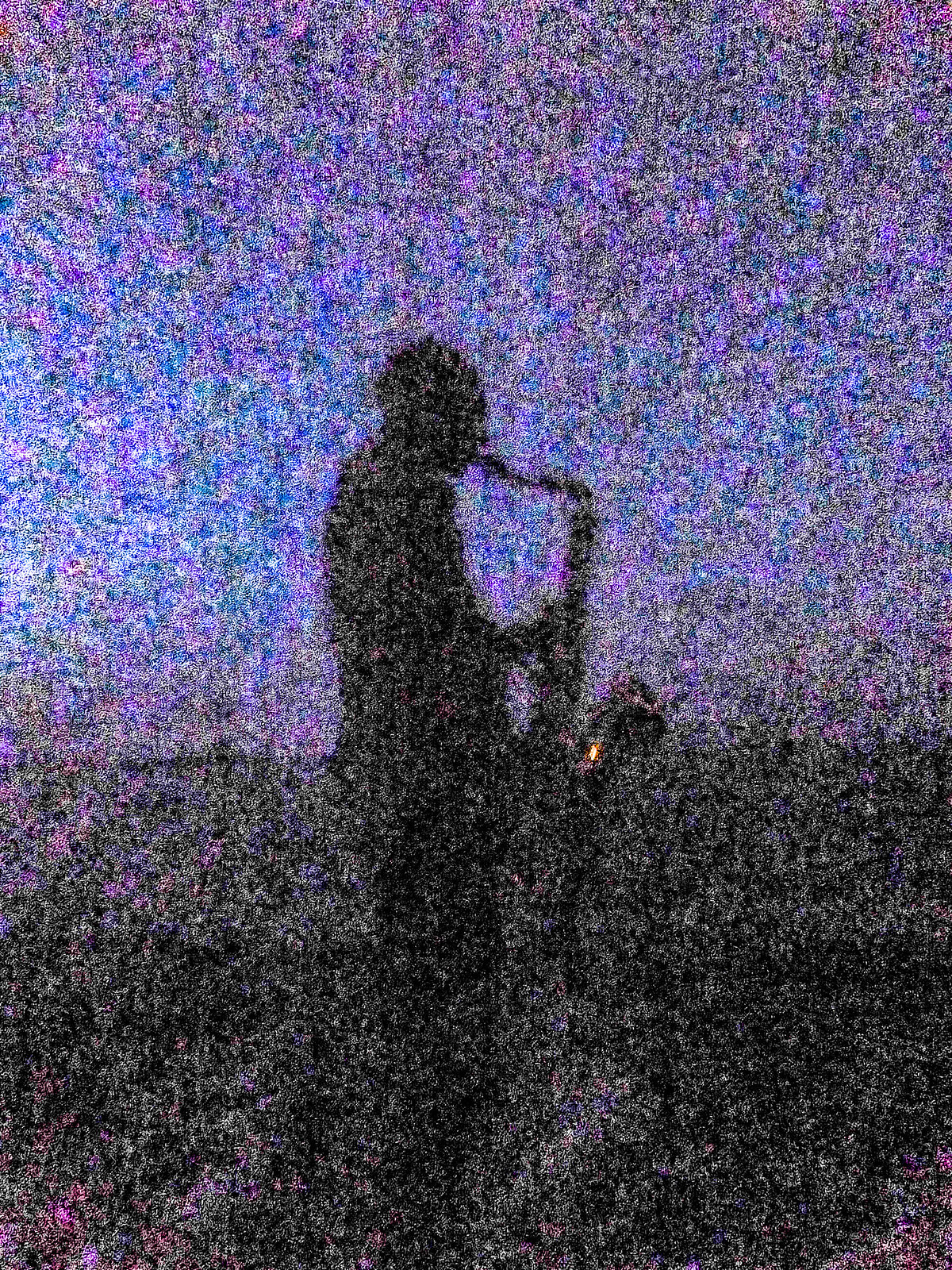The image depicts a heavily pixelated and corrupted photo featuring a silhouette of a man playing a saxophone, likely a tenor saxophone, viewed from a side profile facing to the right. The saxophone itself has hints of gold coloration. The background is divided with the top half displaying retro-styled hues of purple, blue, and green, attempting to replicate a sky, while the bottom half is black or very dark, merging almost indistinguishably with the silhouette. The entire image is plagued with pixelated noise and white snow, making it difficult to discern finer details. The silhouette stands prominently at the center of the image, with the horizon line marking the division between the "sky" and the "ground" positioned at the start of the bottom third of the photo.